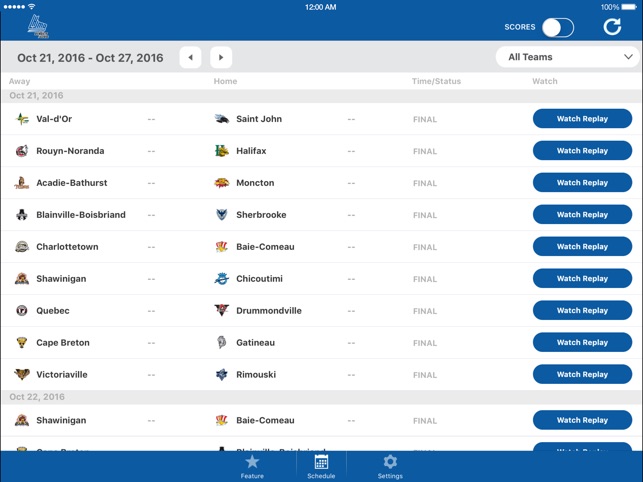This is a detailed screenshot of a web page, likely viewed on a tablet given the wide aspect ratio. The top middle of the screen displays the time as 12:00 a.m., and the top right indicates the device is fully charged at 100%. Directly below the battery icon, there's a score slider feature, which appears to be in the off position, positioned to the left. Adjacent to this is a refresh button characterized by an arrow forming a circular shape.

On the top left, the date range "October 21st, 2016 to October 27th, 2016" is displayed, with navigational left and right arrows to revert or advance the week. 

At the bottom, there's a comprehensive list of names that likely represent different teams, including "Val D'Or," "Blainville," "Boyce Brand," and "Charlottetown." The presence of terms like "final" and "watch replay" suggests that this is a sports-related web page, possibly listing the results or playback options of various matches or games.